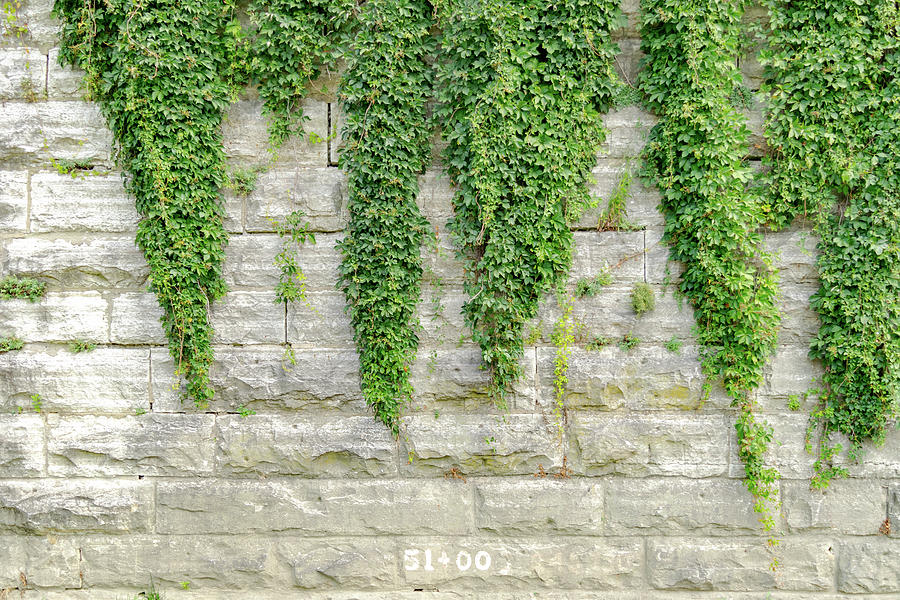This image captures a close-up view of an old, light gray brick wall in horizontal landscape orientation. The weathered bricks showcase many cracks and chips, suggesting age and wear. Descending from the top of the wall are five lush, green clumps of ivy, creating a triangular pattern as they spread downwards. At the bottom middle of the photo, the text "51 + 00" is prominently displayed in white on one of the bricks, though it's uncertain if this is stamped digitally or physical marking on the stone. The vibrant green vegetation against the pale, aged bricks creates a striking contrast, adding a touch of nature to the man-made structure.